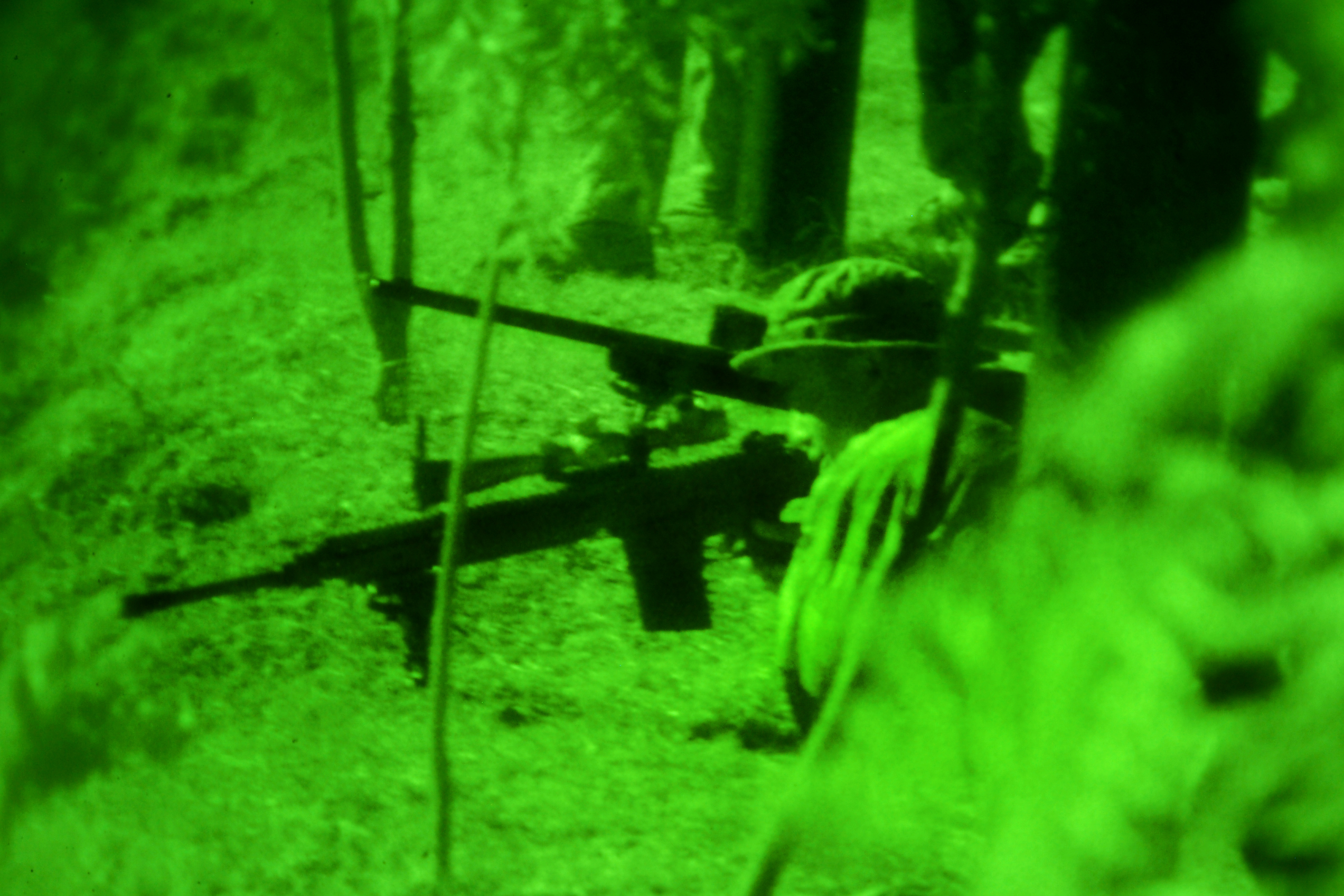This photograph, taken through night vision goggles, captures an intense moment in a forested environment during what appears to be an active combat situation. The image, rendered in green and black, shows a soldier wearing a canvas-style hat and a long-sleeved shirt or jacket that blends into the surrounding vegetation. The soldier is seen leaning on his elbows on the ground, intently aiming a long-barreled automatic weapon with a prominent scope towards the left of the frame. Beside him, partially obscured by his body, the barrel of another gun protrudes, indicating the presence of a second person similarly poised and aiming in the same direction. Thin trees and dense foliage surround them, further enhancing the clandestine, high-stakes atmosphere of the scene. The grainy texture and the green filter, reminiscent of a heat sensor or night vision effect, underscore the urgency and tension of the moment.